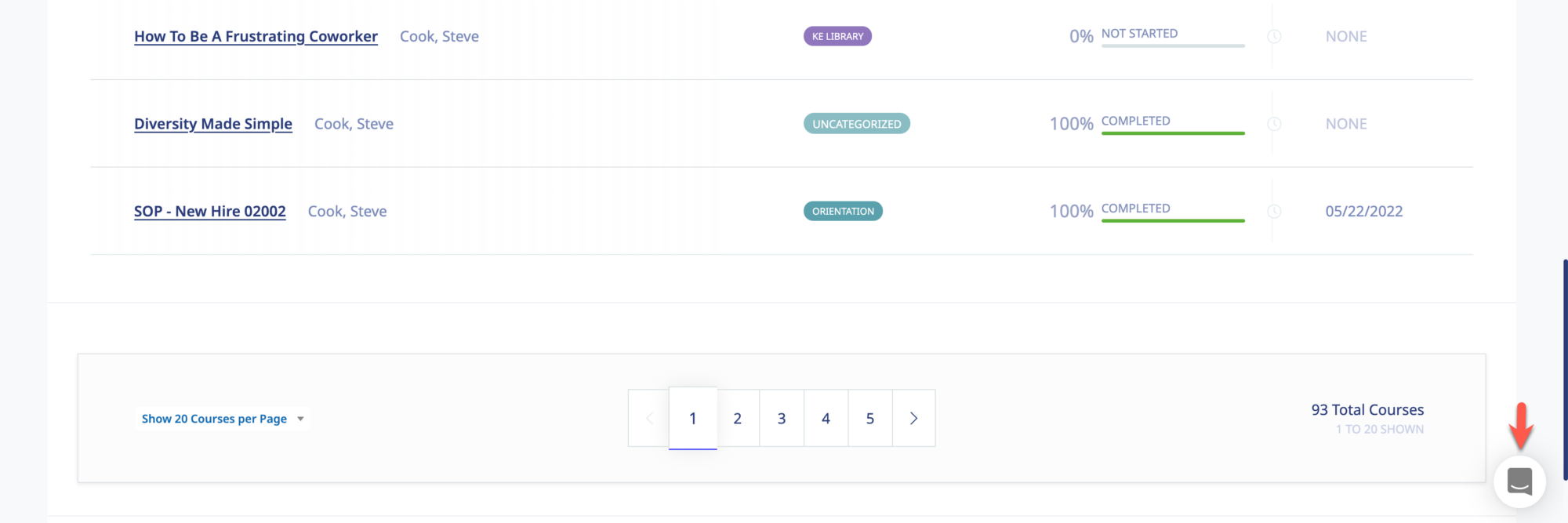This image is a digitally altered screenshot from a course provider's website, marked to highlight specific content. A red arrow has been added to the bottom right corner, pointing towards the messages hub, likely indicating where users can find support or additional information. 

The website in question offers a wide array of courses, as evidenced by the note at the bottom of the screenshot, which states there are 93 total courses spread across pages 1 to 20, with the current settings displaying 20 courses per page. 

Highlighted within the screenshot are three courses:
1. **"How to Be a Frustrating Co-worker" by Steve Cook** - This course has not yet been started by the user.
2. **"Diversity Made Simple"** - This course is 100% complete.
3. **"SOP New Hire 02002" by Steve Cook** - Also fully completed, with completion marked as part of the user's orientation on May 22, 2022.

This screenshot has potentially been submitted by a customer services team to illustrate the possibilities of post-original capture editing and to help guide users on where to access support.